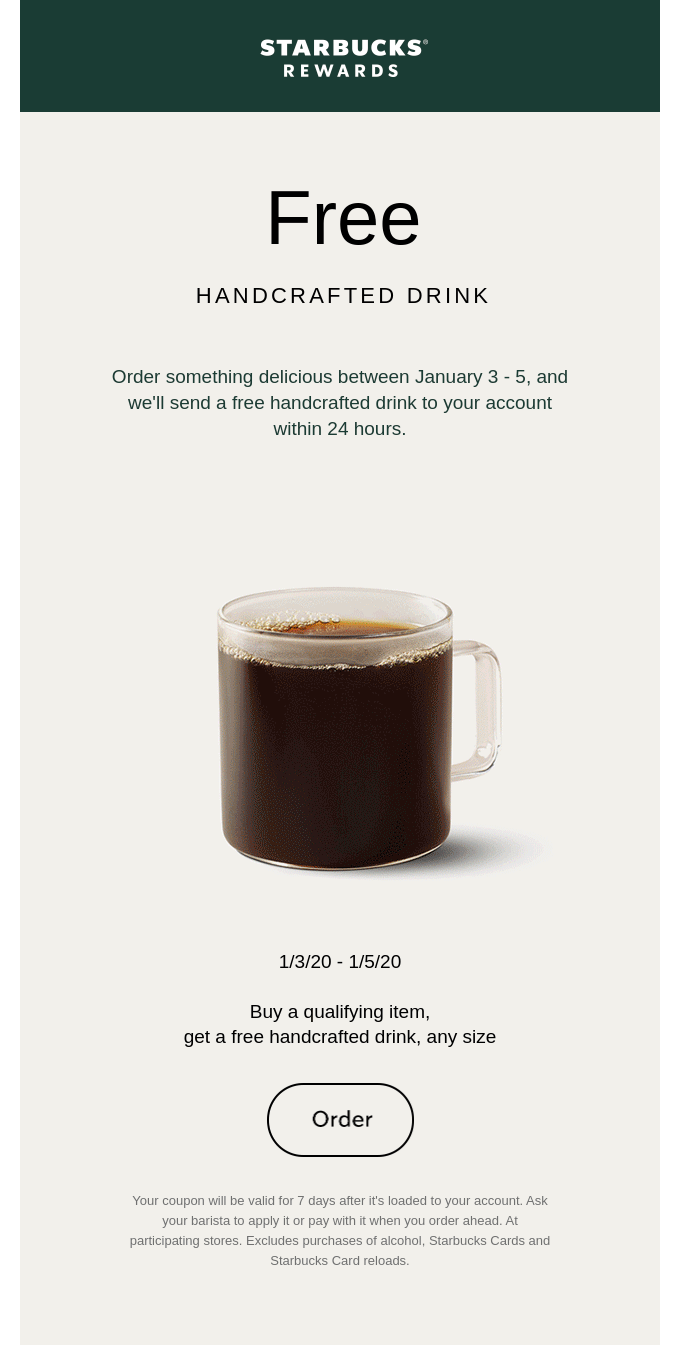Detailed Caption: 

A screenshot from the Starbucks Rewards app displayed on a smartphone showcases a promotional offer set on January 3rd through 5th. At the top of the screen, the 'Starbucks Rewards' header is in white text against the signature dark green background. Dominating the center of the image, the largest text reads "FREE," highlighting the main appeal of the promotion: a complimentary handcrafted drink. The offer encourages users to "order something delicious," specifying that upon purchase of a qualifying item, a free handcrafted drink will be credited to their account within 24 hours. 

Accompanying the text is an image of a clear coffee mug devoid of any logos, filled with coffee. The mug's handle is oriented to the right, drawing attention to its simplicity. Additional details explain that the complementary handcrafted drink can be of any size. A circular button labeled "Order" is prominently featured, inviting users to take action. The final note confirms that the coupon for the free drink will be valid for seven days after being loaded into the user's account. All of these details are aggregated at the bottom of the screen, providing a comprehensive view of the offer.